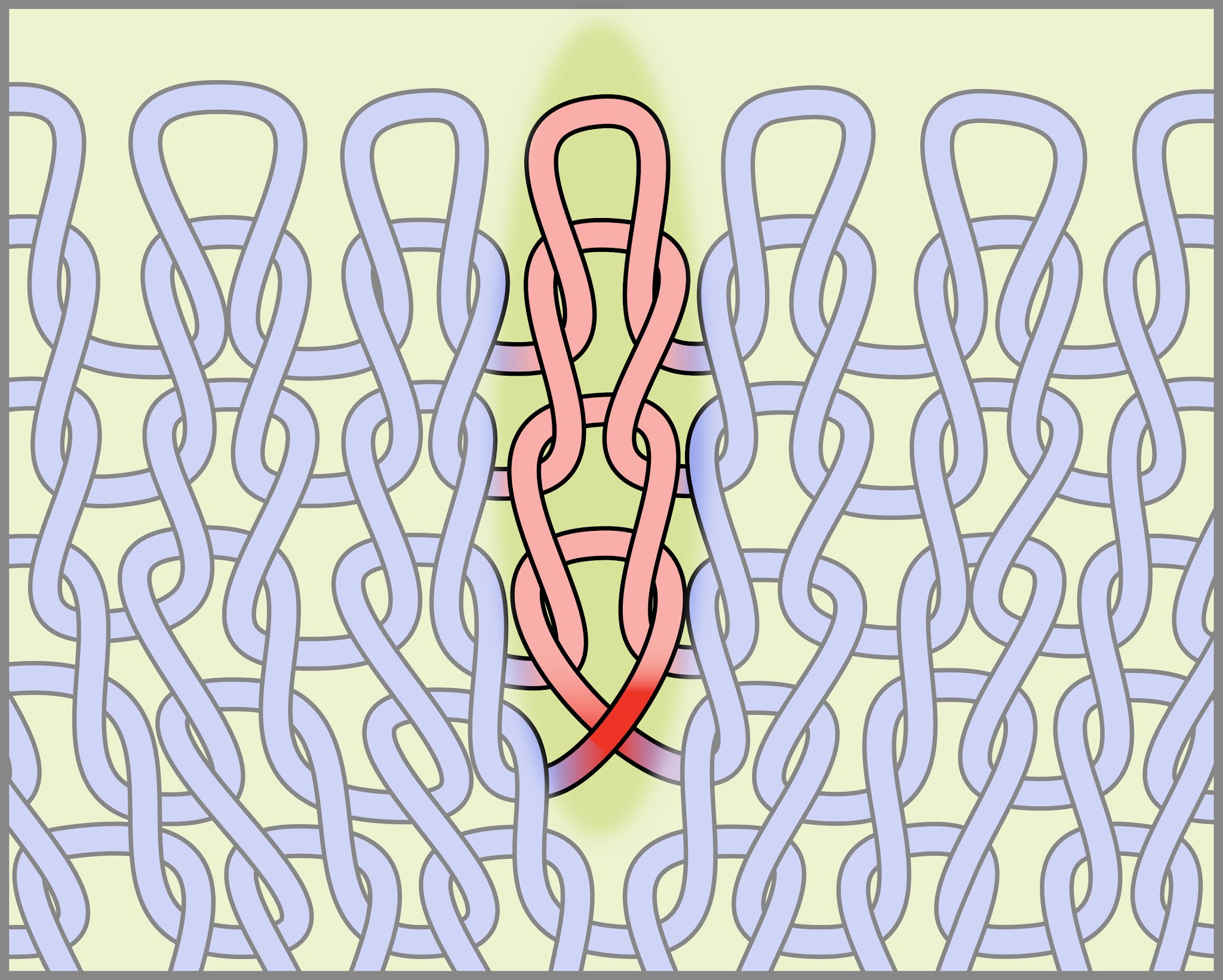This image is a detailed graphic featuring a series of interlinked elements, resembling chain links, arranged in a grid with six columns and four rows. Most of the links are baby blue with dark gray perimeters, creating a harmonious and repetitive pattern. The central column stands out, displaying links that transition from pink at the top to bright red at the bottom, and these links have a black perimeter. The background is primarily a light gray, but shifts to green behind the pink and red links in the middle column. The overall pattern of the links moves diagonally, going from left to right, downwards, upwards, and then repeating. This cartoon-like drawing is visually abstract with no accompanying text, and features a color palette that includes black, white, various shades of blue, purple, red, pink, and green.